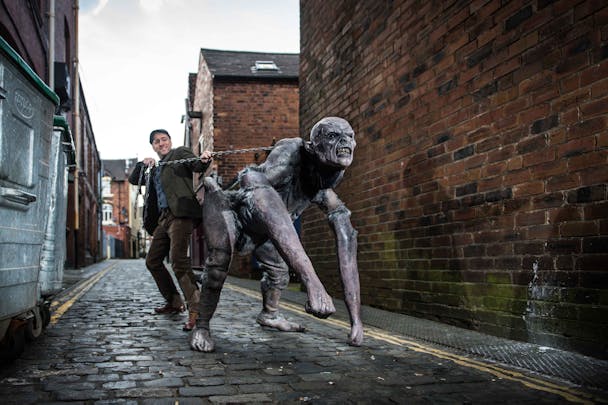The image is a screenshot from a movie, featuring a mix of live-action and CGI elements to create a fantastical scene set in a narrow alleyway. The alleyway is paved with dark brick pavers marked by double yellow lines on either side. Surrounding the scene are red brick row houses that evoke the atmosphere of an old European city, possibly London or Ireland. 

In the center of the image stands a young man with Caucasian skin, wearing a flat cap, a green jacket over a blue shirt, and brown pants. His coat is opened at the front, revealing a light-colored waistcoat. The man is engaged in pulling a metal chain connected to a monstrous creature that appears to be a hybrid of human, zombie, and werewolf features. 

The creature has a bald, gray head with a snarling, demonic face that shows bared teeth. Its body is thick and wide, covered in patches of fur at the shoulders, and it wears pants but no shoes. The creature’s elongated arms drag on the ground, resembling a human's but much longer and with clubbed fists. Its feet are similarly distorted, half-human, and ending in long claws. Additional details that lend an eerie, unsettling tone include the creature's hip bones jutting outward and its overall menacing posture as it looks down the alleyway. The ground to the right features a gray garbage bin on wheels, further grounding the surreal scene in a mundane, urban setting.